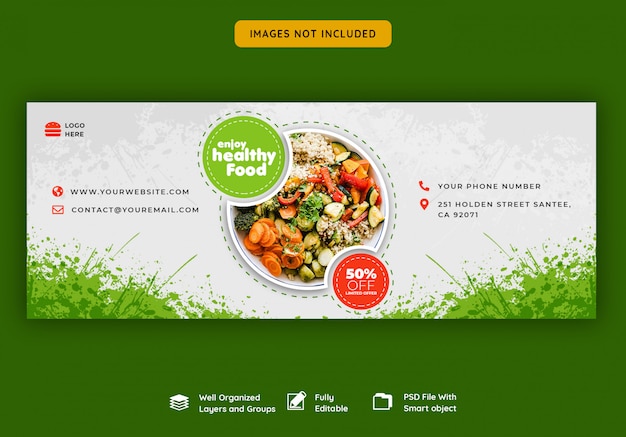The image is a webpage template featuring a green background. At the top of the page, a yellow text box with the message "Images not included" is prominently displayed. Beneath it, another text box marked "Logo Here" contains a red hamburger icon, accompanied by the phrase "Enjoy Healthy Food."

The focal point of the webpage is a centrally positioned circular plate brimming with an assortment of vibrant vegetables in hues of green, orange, red, and other colors. Adjacent to this plate is a red circular icon stating "50% Off, Limited Offer."

On the right-hand side, the webpage template includes the following contact details:
- Website: yourwebsite.com
- Email: contact at youremail.com
- Phone number: [Insert your phone number]
- Address: 251 Holden Street, Santee, California, 92071

At the bottom of the template, there's a note that reads, "Well-organized layers and groups, fully editable, and a PSD file with a Smart Object."

Overall, this webpage template offers a visually appealing and organized layout suitable for businesses looking to promote healthy food options. The green background and the vibrantly colored food imagery make it an inviting choice for companies aiming to showcase fresh, healthy products.